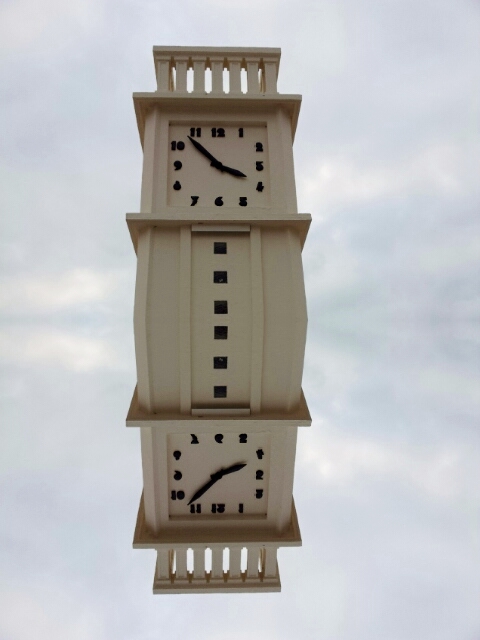The photograph showcases a captivating and artistic rendering of a clock tower structure that appears mirrored both in the top and bottom halves of the image. Each half features a white, clay-colored tower with a square-shaped black-and-white clock. The clocks, set to approximately 3:54 PM, have two thin hands—a short hand near the floor and a longer hand almost touching the 11. This reflective symmetry gives the impression that the bottom of the image is an inverted copy of the top. The tower is adorned with three small window slots toward the center and is flanked at the top by a row of six or seven small stone columns. Surrounding the structure, the background consists of a light bluish-gray sky dotted with wispy, articulated clouds. The artistic nature of the piece creates an illusion of the clock floating in an ethereal, cloud-filled space.